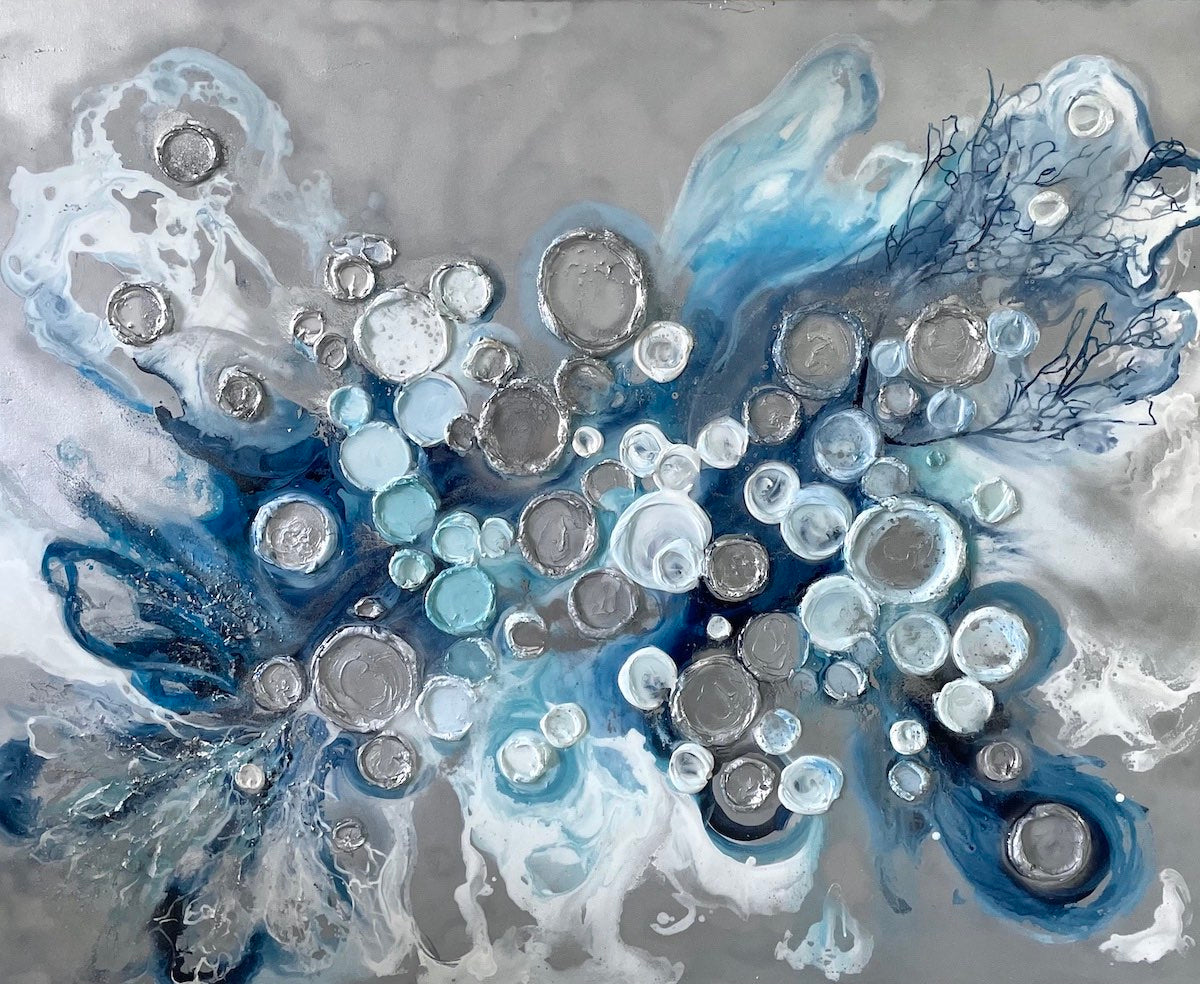The artwork depicted in this wide horizontal image appears to be an abstract oil painting, featuring a dynamic blend of colors and shapes. Dominating the background is a slate grey and white base, interspersed with a variety of blue shades ranging from dark, almost teal-like blue to a cool ocean blue. This grey background has a slightly shiny, silvery quality that catches the light, adding a layer of depth and texture. 

Centrally, the painting showcases a myriad of swirling shades and patterns that evoke the fluidity of raindrops on still water or the pockmarked surface of the moon. These swirls culminate in a striking middle section with splatters and drops in silver and white, mingling with the blues to create a visually captivating focal point. Amidst this chaotic yet harmonious center, dark blue lines appear, veiny in their arrangement, suggesting the delicate outlines of flowers or the wings of a butterfly.

In terms of composition, the image is framed by abstract, waving patterns of paint that seem to cascade and drip across the canvas, enhancing the overall sense of movement. Accentuating these flowing forms are detailed, black branch-like decorations in the upper right corner and white leaf motifs in the bottom left, adding a touch of organic intricacy to the piece. 

Despite its abstract nature, the painting is both stark and alluring—appearing as a complex interplay of color, texture, and form that makes it a compelling, albeit somewhat generic, stock image of modern art.